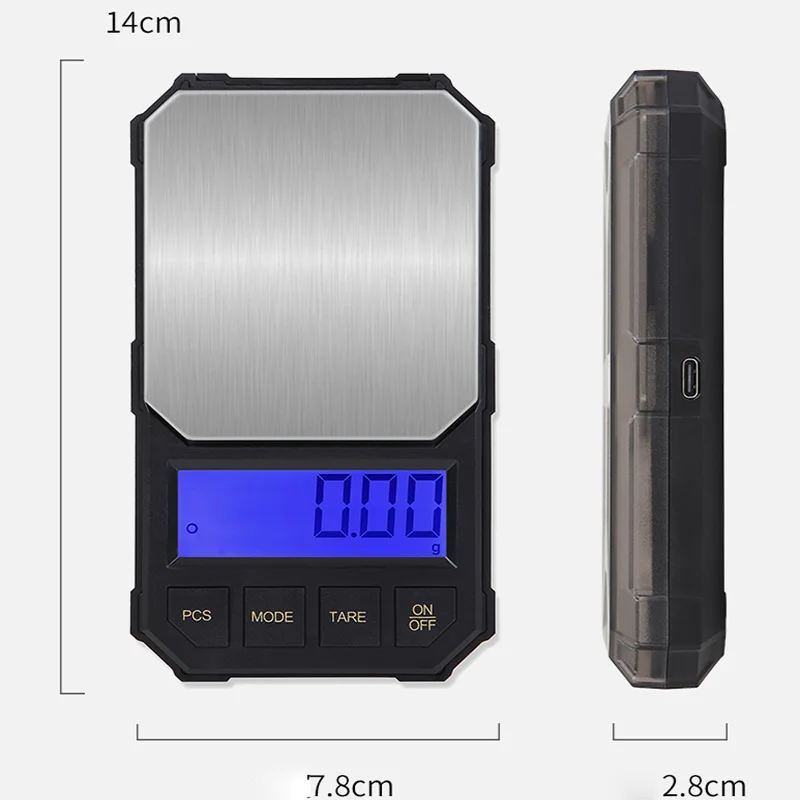This image displays a small digital scale against a white background, featuring two different perspectives. The left side shows an overhead view, revealing a rectangular scale with a silver weighing plate bordered by black plastic. Prominently, a blue digital screen with black lettering reads "0.00 grams." Beneath the screen, four gold-colored buttons are labeled (from left to right): PCS, Mode, Tare, and On/Off. The right side of the image provides a side profile, highlighting a charging port and indicating the dimensions as 14 centimeters in height, 7.8 centimeters in width, and 2.8 centimeters in depth. This compact scale, designed for precise measurements in grams, is likely intended for tasks such as mailing or cooking.